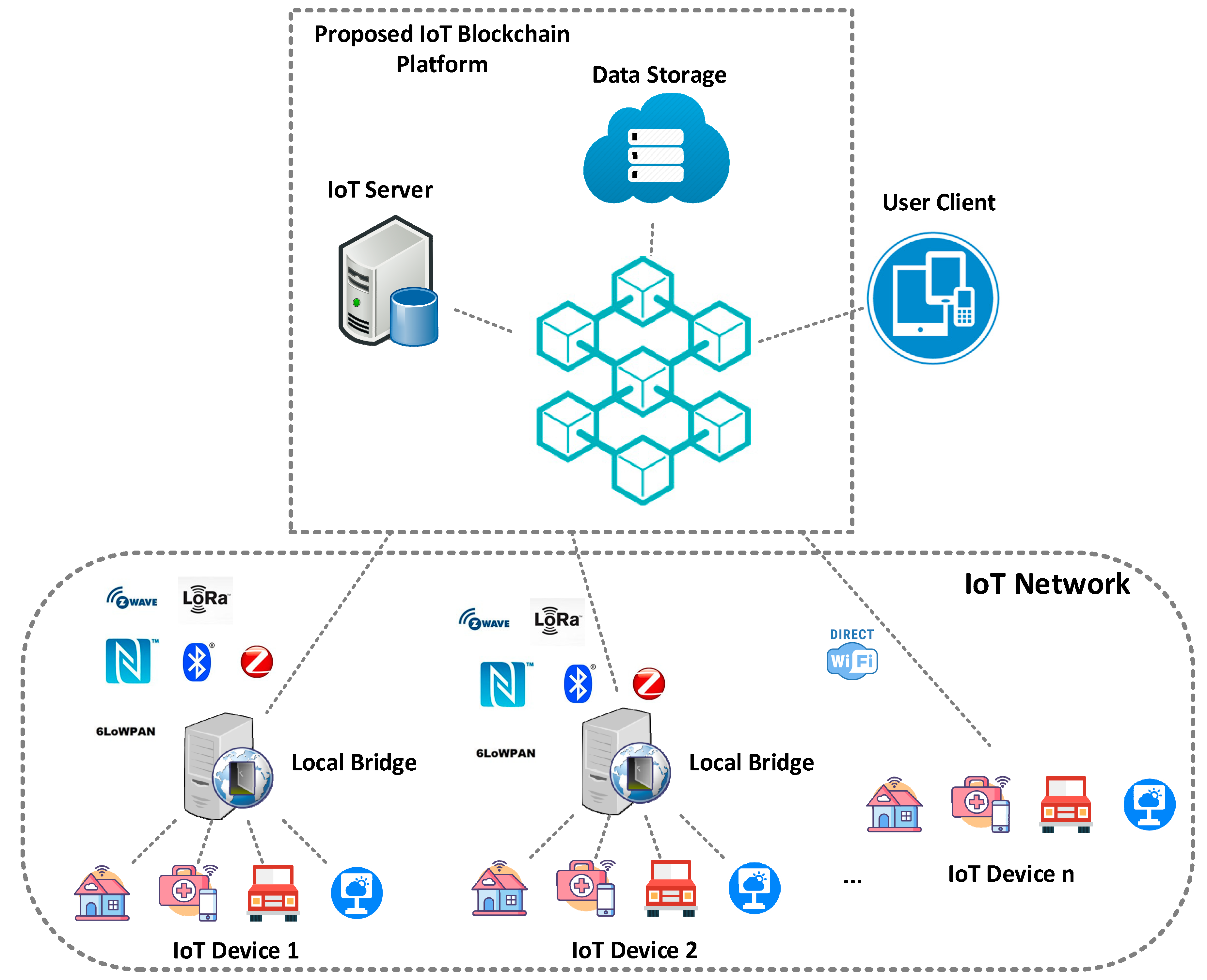The image is a detailed illustration of a proposed IoT blockchain platform, divided into two main segments. The top segment features a square with a white background and a gray dotted outline. In the upper left corner of the square, the text "Proposed IoT blockchain platform" is inscribed in black. Within this square, there's a smaller gray server icon labeled "IoT server," resembling an old desktop computer with a white circle adjacent to it. Positioned to the top right of the server, the term "Data Storage" appears alongside a blue cloud containing three right rectangles. These elements are interconnected with teal blue bars forming a grid of seven small, teal-colored cubes. Extending from this grid is a line pointing to another element identified as "User Client," encompassing icons of an iPad, cell phone, and another possible tablet within a medium blue circle.

The bottom segment displays a more complex, horizontally-oriented rectangular diagram with curved edges, labeled "IoT Network" in the upper right corner. Three lines link the upper square to this lower rectangle. On the left side, labeled "Local Bridge," there's an image of a desktop computer with four lines extending to icons of a house, a medical briefcase with a cell phone next to it, a red car viewed from the front, and a circular blue icon with a white monitor. The mid-section and right side of this rectangle feature identical sets labeled "IoT Device 1," "IoT Device 2," and "IoT Device N," highlighting that the lower segment can represent an indefinite number of IoT devices, each including the house, briefcase, car, and monitor illustrations.